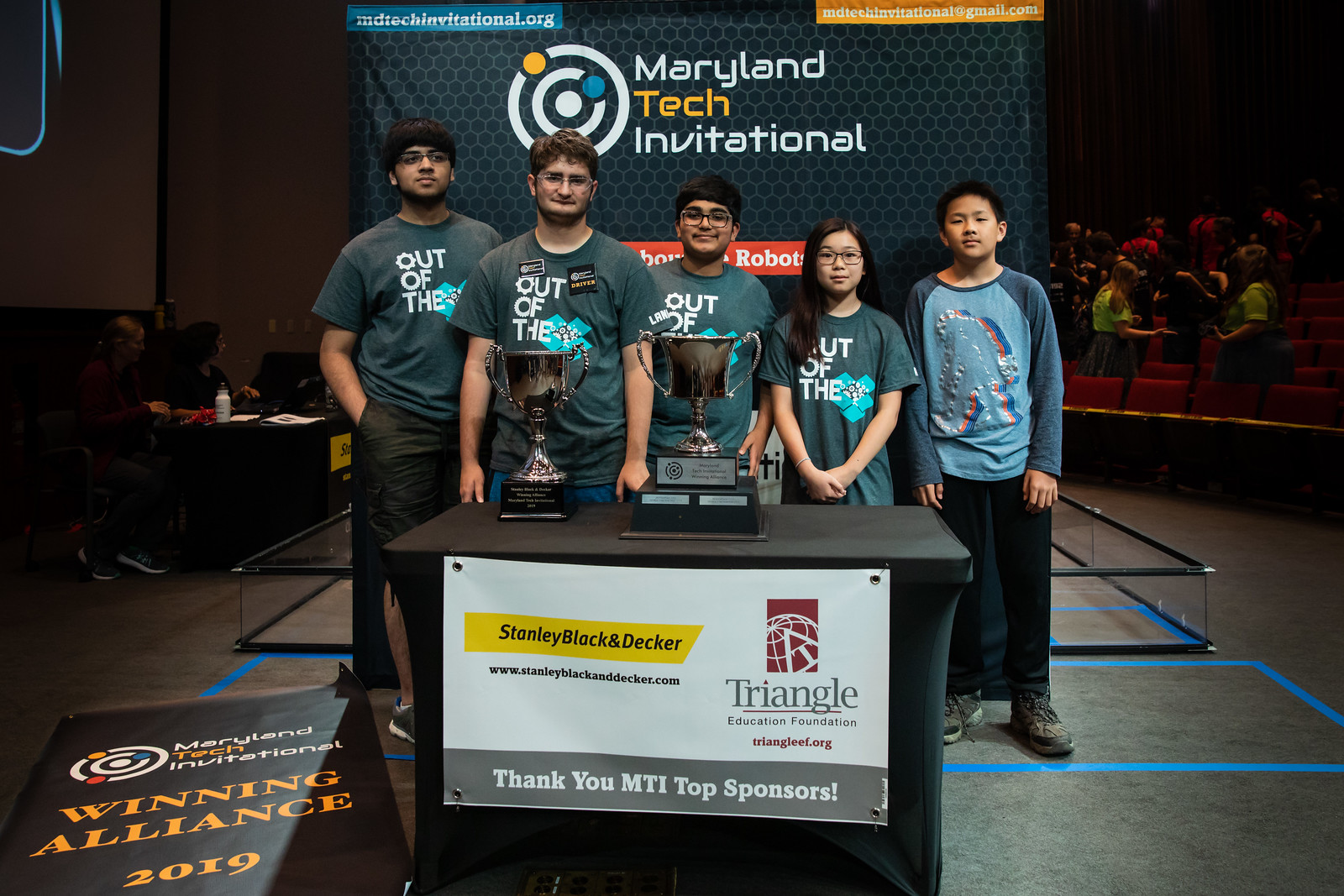The image depicts a scene from the Maryland Tech Invitational where five individuals, presumably students, are standing at the center, gradually dominating the frame. Four of them, likely boys, and one girl, are wearing shirts with an "Out of the Box" slogan, except for one person wearing a shirt with a rainbow design. Behind this group is a table adorned with trophies and a sign proudly announcing "Stanley Black & Decker Triangle Education Foundation Thank You MTI Top Sponsors." The Stanley Black & Decker logo, characterized by its black and yellow palette, along with the Triangle Education Foundation logo in red and gray featuring a red square with a globe, are prominently displayed. A backdrop banner reads "Maryland Tech Invitational Winning Alliance 2019." In the background, there are additional people at a black desk, including two women in red and black attire. The crowd is seated in an auditorium-like setting with gray floors and red chairs. The indoor venue's warm color palette includes tones of tan, brown, maroon, yellow, red, blue, white, and gray, indicating it’s a vibrant and dynamic event space designed for this tech competition.